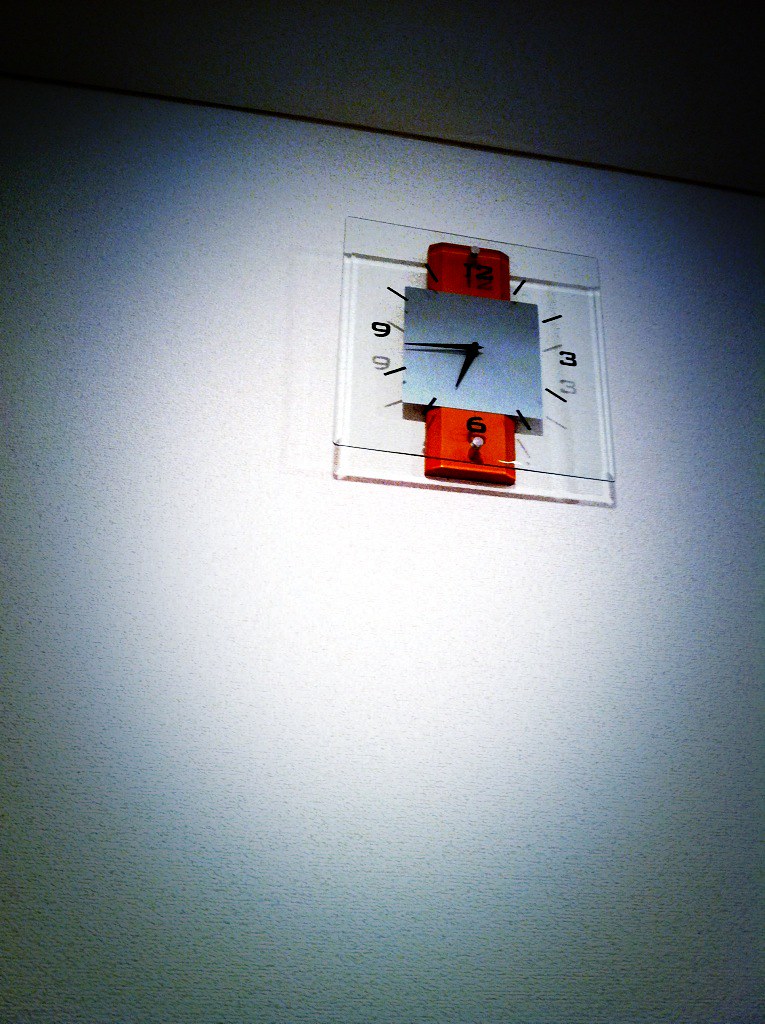The indoor color photograph captures an upward-looking view of a clock mounted on a white wall, depicted from a slight angle. The clock features a square shape and appears to be made from transparent material, either glass or plexiglass, allowing the wall behind it to be partially visible. Only the numerals 12, 3, 6, and 9 are displayed prominently, with hash marks representing the other hours. The time displayed is approximately seventeen minutes past six. At the center of the clock face is a steel-colored square, anchoring the clock's hands. Behind this central element, a vertical, reddish bracket can be seen, likely securing the clock to the wall. Subtle light reflections project the numerals onto the wall, enhancing the ethereal quality of the scene. The image is characterized by darker tones in the upper and lower corners, creating a vignette effect that adds depth to the composition.